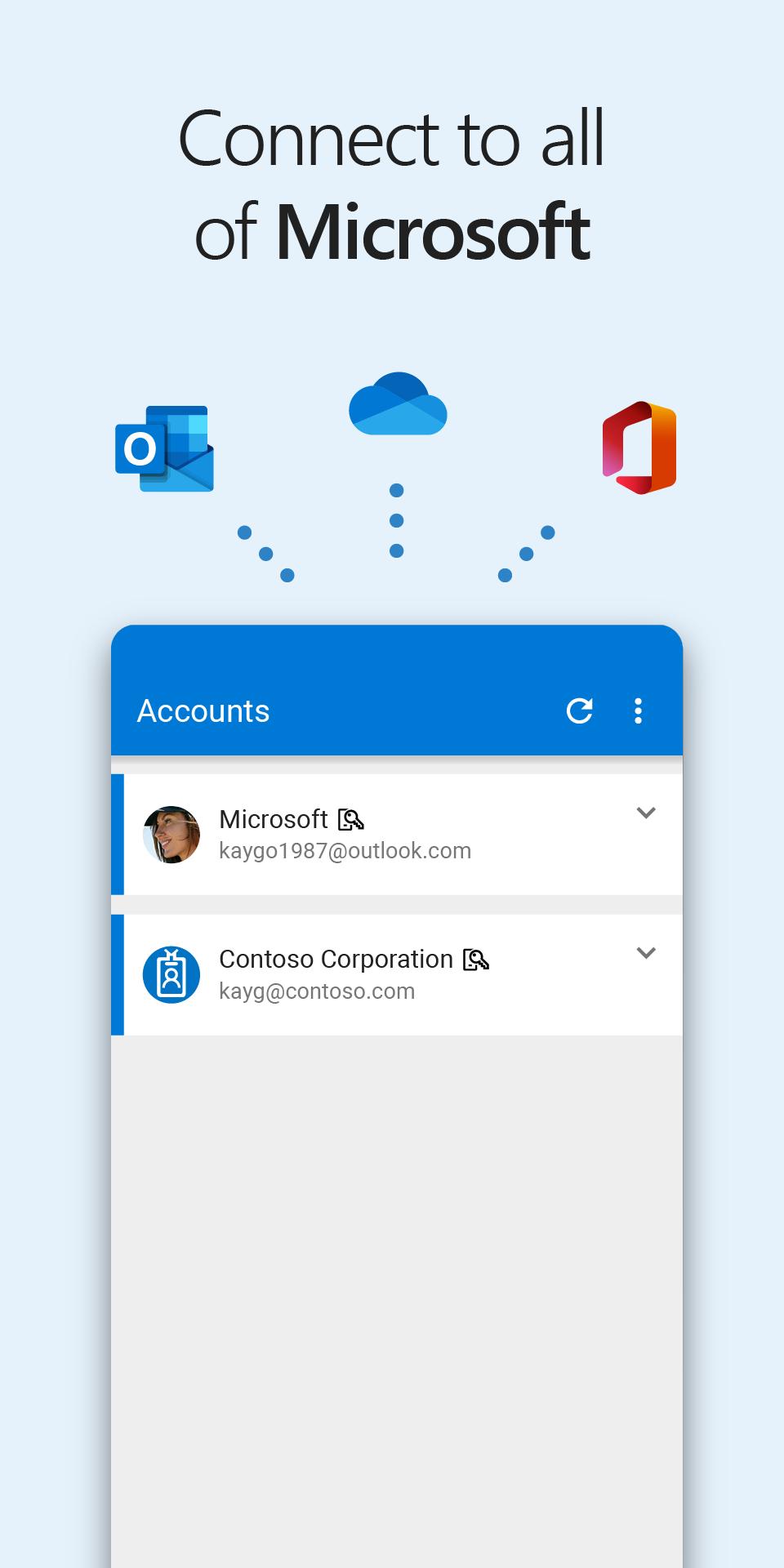The image has a light blue background. About an inch from the top center, the word "CONNECT" is prominently displayed in capital letters. Below this, still centered, is the phrase "to all." 

Underneath "to all," the term "of Microsoft" is written, with "Microsoft" in bold capital letters. 

Beneath these texts, there is an illustration of a blue cloud. The cloud is dark blue on the top, light blue on one side, and medium blue on the other sides, with three blue dots aligned vertically descending from it. 

To the right of the cloud, there is a red square, slightly rotated to show its right side towards the camera, with three blue dots descending to its left. 

On the far right, an email icon is visible with a small piece of blue paper peeking out of the top. 

Adjacent to this icon, there is a little square on the left that contains a white circle with three blue dots aligned vertically to its right. This section has a blue border about an inch wide on the left side and features the word "accounts."

On the right side of this section, there are three ellipses aligned vertically, followed by a refresh button to their left. All elements are rendered in white with a thin gray border surrounding them.

Additionally, there is a white tab with a blue border running across its left side. The tab displays a profile picture of a girl on the right side with the text "Microsoft" adjacent to it. Underneath the name, the email address "KGO1987@outlook.com" is written. To the right of this tab, a greater than sign is pointing down.

Below, there is another white tab with a similar blue border on the left. This tab features a blue circle containing a small square and a profile icon. The text "Contoso Corporation" is mentioned next to the blue circle. Underneath, it lists the email address "KG@Contoso.com."